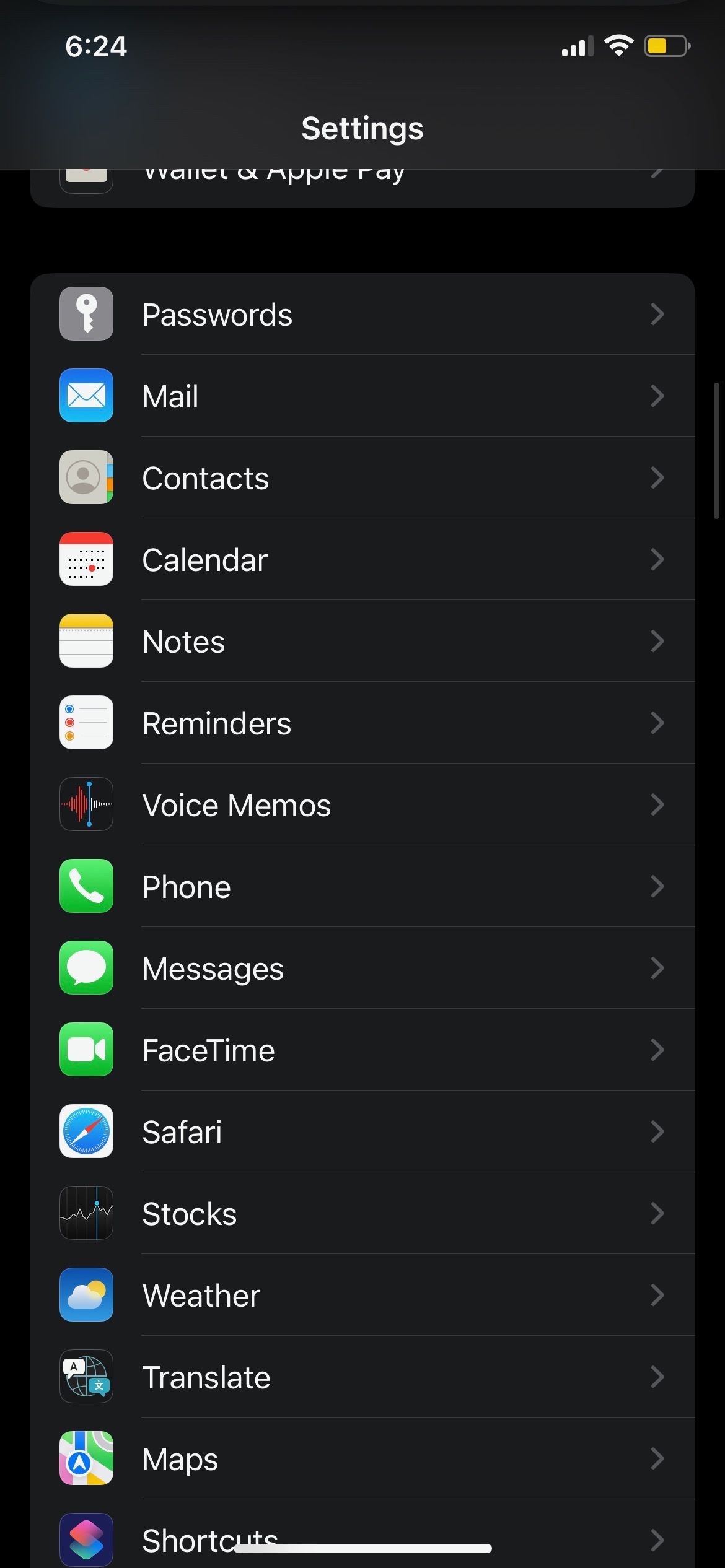In this image, we observe a screenshot captured from a cell phone. The background is predominantly a solid black shade, with some areas appearing as a dark charcoal gray. A black header runs across the top of the screen. In the upper left corner, white text displays the time as "6:24." The upper right corner features three icons: the reception signal with three out of four bars lit, an activated Wi-Fi symbol, and a battery icon indicating it is half full.

Prominently central in large, bold white text is the word "Settings." Right below, a partial view of "Wallet & Apple Pay" is visible. The main portion of the screenshot showcases a series of icons accompanied by text labels. These are sequentially arranged as follows:

1. "Passwords" accompanied by an icon of a key.
2. "Mail"
3. "Contacts"
4. "Calendar," represented by a white icon with a red top banner.
5. "Notes"
6. "Reminders"
7. "Voice Memos"
8. "Phone"
9. "Messages"
10. "FaceTime"
11. "Safari"
12. "Stocks"
13. "Weather"
14. "Translate"
15. "Maps"
16. "Shortcuts"

The combination of icons and text gives the screenshot a structured and organized appearance, typical of a smartphone settings menu.